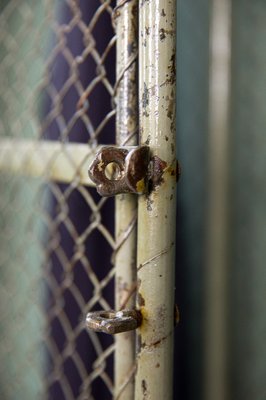This detailed portrait image depicts a section of a chain-link gate against a muted background primarily colored in green, brown, and black. The gate features several metal bars, with one prominent bar rising straight up the center and another bar attached to a chain-link fence situated next to it. Another bar extends from the center towards the left-hand side, while a fourth, more blurred bar can be seen emerging on the right-hand side. The poles, painted a chipped brownish-gray, show signs of aging with visible rust spots. Additionally, a bracket is welded to the end of one of the bars, and a latch mechanism is visible, indicating where the gate might lock. The chain-link fence itself is silver and attached to these aging, rust-spotted bars. The partially visible background reveals either a light green wall or section of the wall, further emphasizing the worn and rustic aesthetic of this gate section.